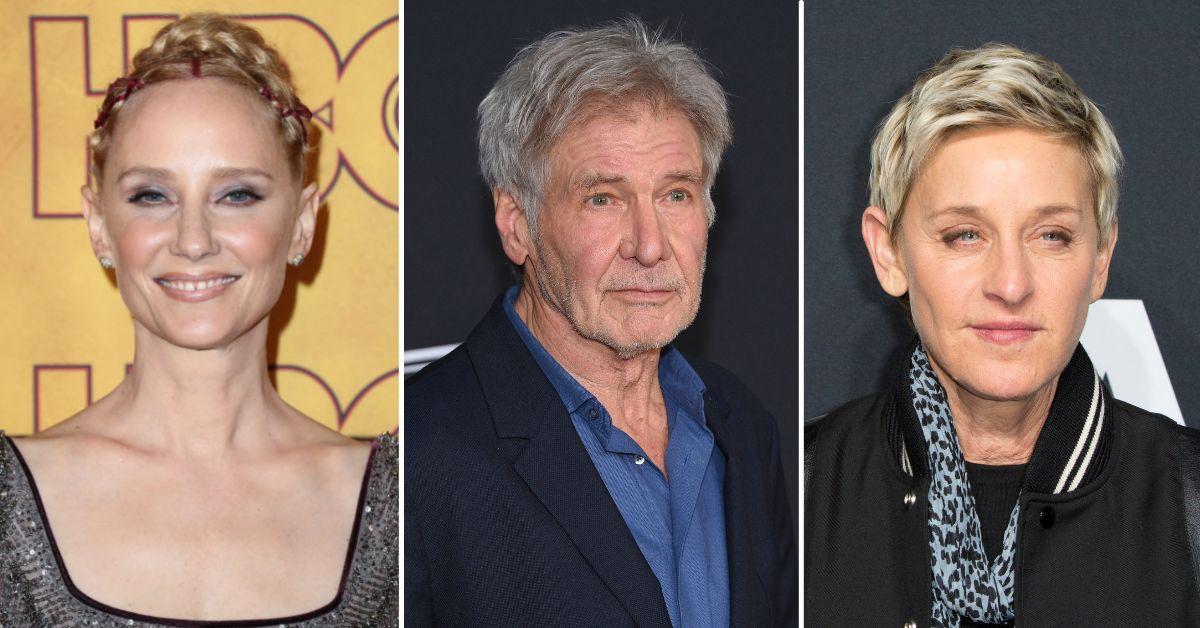This image showcases three celebrities, each in a separate frame. On the left is a woman with blonde hair styled in an elaborate updo, possibly Celine Dion, Sarah Jessica Parker, or Anne Heche. She stands smiling against a yellow background with "HBO" printed in black outline. She is wearing a sparkling black, square-necked top adorned with sequins and accessorized with earrings. In the center, Harrison Ford looks directly at the camera with a slightly tired expression. He sports gray hair, light stubble, and is dressed in a plain blue button-up shirt under a blue jacket. On the right is Ellen DeGeneres, also looking into the camera without a smile. She has short, cropped blonde hair and wears a sporty jacket with a black and white striped collar, paired with a blue and black leopard print scarf. Each celebrity appears to be in a different setting and not interacting with one another.